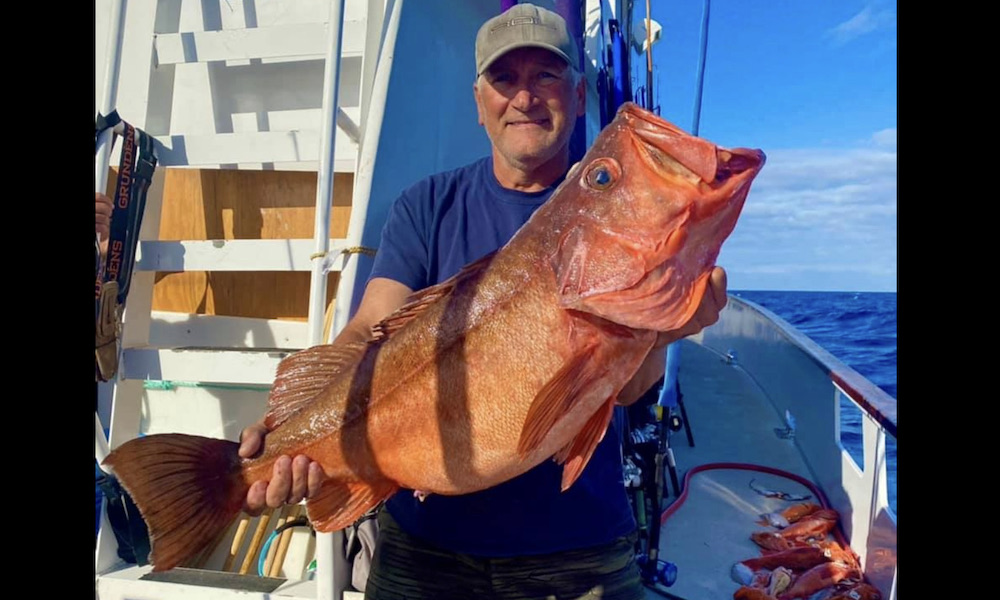A man, likely Caucasian and older with white hair, stands proudly on the deck of a fishing boat, holding a large red grouper he just caught. He is dressed in a blue short-sleeved shirt, faded green baseball cap, and camo pants. The man, who has no facial hair, holds the fish out in front of him with one hand gripping just below the tail and the other hand supporting under the gills, showcasing its impressive size—nearly spanning the width of his body. The red grouper's leather-like, red appearance is striking against the background. The scene is set in the middle of a calm, blue ocean under a sky dotted with a few white clouds. The boat's deck features scattered fishing tackle, poles, and other caught red groupers. A white-painted wall outlines the edge of the boat, with a stairway leading to a higher deck visible on the left and possibly another person's hand in the background. The overall image captures the triumphant moment of a successful fishing trip.